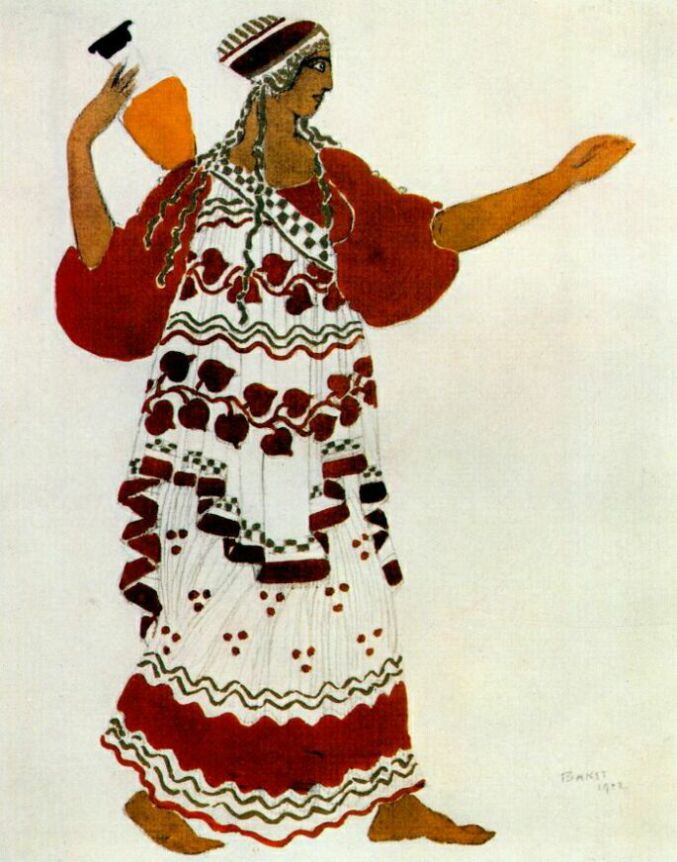The painting depicts an Egyptian-looking woman with dark brown skin, who is barefoot and standing sideways, carrying a transparent urn with orange liquid and a black lid on her left shoulder. She wears an elaborate red and white dress that extends to her ankles. The dress features elbow-length, puffy red sleeves, and a white sash adorned with a leaf pattern in burgundy, red, and purple. The lower part of the dress is decorated with intricate designs, including red wavy stripes flanked by dark green lines and polka dots. Her hair is styled in dreadlock-like braids cascading down, and she wears a hat that's primarily red with black and gray accents, as well as green stripes at the top. The background is a stark white wall with an indistinct signature and date that appears to be 1903.